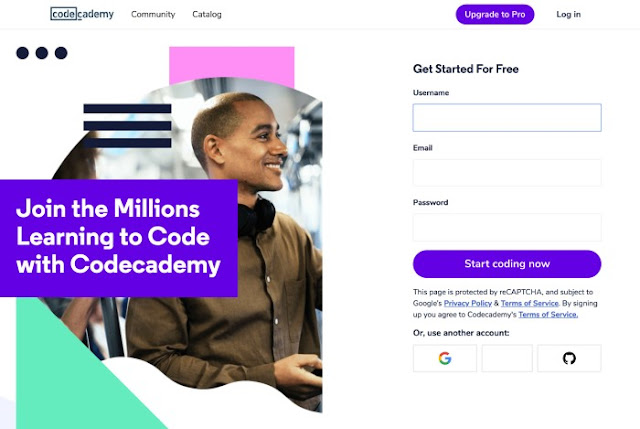This image depicts a sign-up page for learning coding through Code Academy, prominently labeled "Code Academy Community Catalog" in the top left corner. On the upper right, there are clickable options reading "Upgrade to Pro" and "Log In." Below these, a call to action on the right side of the page invites users to "Get Started for Free." 

The sign-up form includes fields for "Username," "Email," and "Password," each followed by a corresponding blank text box. At the bottom of the form, a prominent button reads "Start Coding Now." The page highlights that it is protected by ReCAPTCHA and subject to Google's Privacy Policy and Terms of Service, noting that by signing up, users agree to Code Academy's Terms of Service or can use another account. There are three additional boxes: one with the Google symbol, another blank, and a white box with a black symbol.

On the left side of the page, there is a photo of a smiling African American young man. Overlaid on this photo is white text on a blue rectangular background that reads, "Join the Millions Learning to Code with Code Academy." Directly below this, a teal or aqua symbol occupies part of the lower left-hand corner of the page.